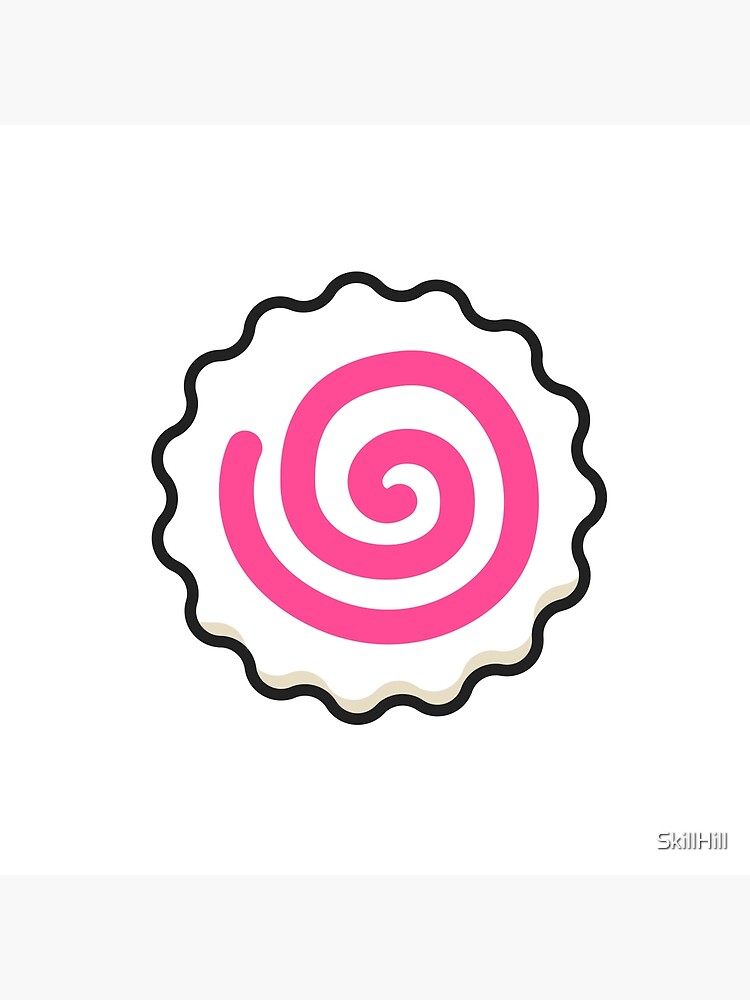The image features a simple, circular design set against a pristine white background, which is letterboxed with light gray areas above and below. At the heart of the design is a black, wavy line forming a cog-like or cookie-shaped outline with small, rhythmic waves—evoking half circles—that encapsulate the piece. This line also features a subtle gray drop shadow, giving it a slight 3D effect. Inside this black-lined perimeter, a bold, hot pink line spirals out from the center in a clockwise pattern, occupying much of the inner space and stopping near the left-middle section of the design. In the lower right-hand corner, there is text in white with a black outline that reads "Skill Hill."